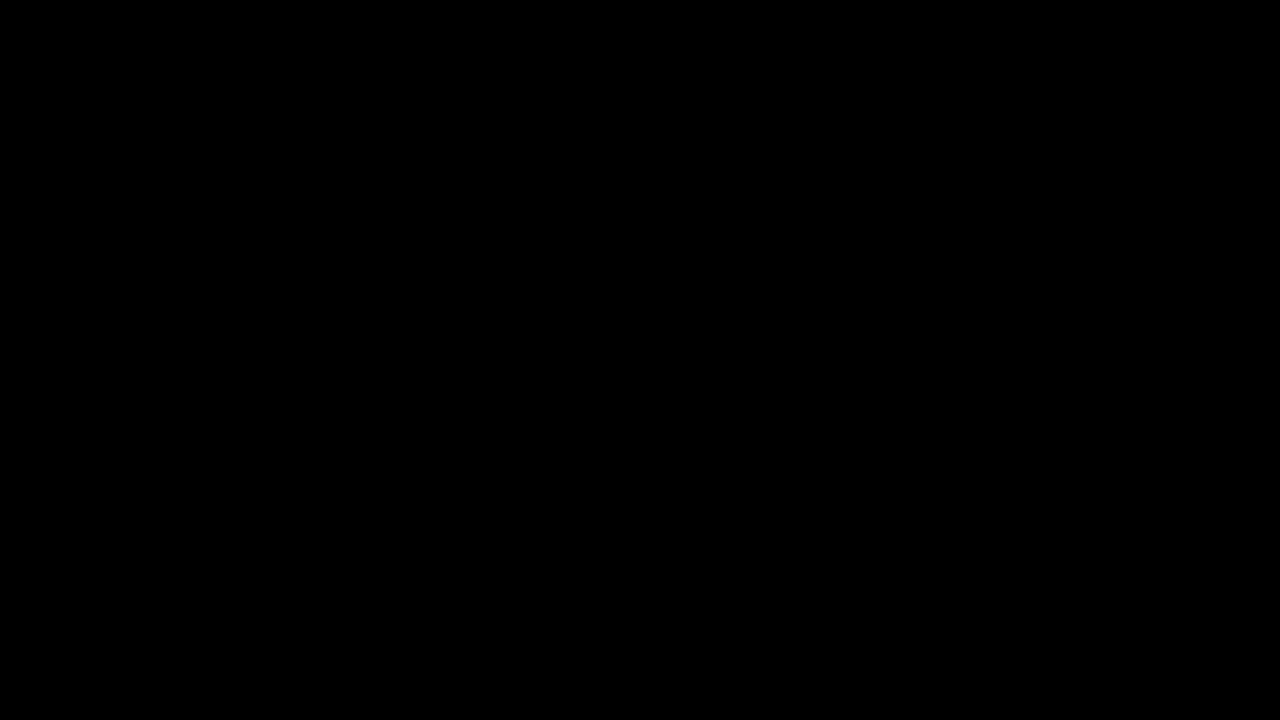The image depicts a completely black rectangle set against a sharp white background, aligned in landscape orientation. The black rectangle is about one and a half times wider than it is tall, with exact proportions showing a width approximately 1.5 times the height. The rectangle features precise, sharp corners without any curvature, and the blackness within it is a deep, uniform shade, with no gradients, textures, icons, or any other graphic elements. The image is purely a solid black box, void of any detail, imagery, or color variations, offering nothing to engage the viewer's attention beyond its stark, minimalist form.